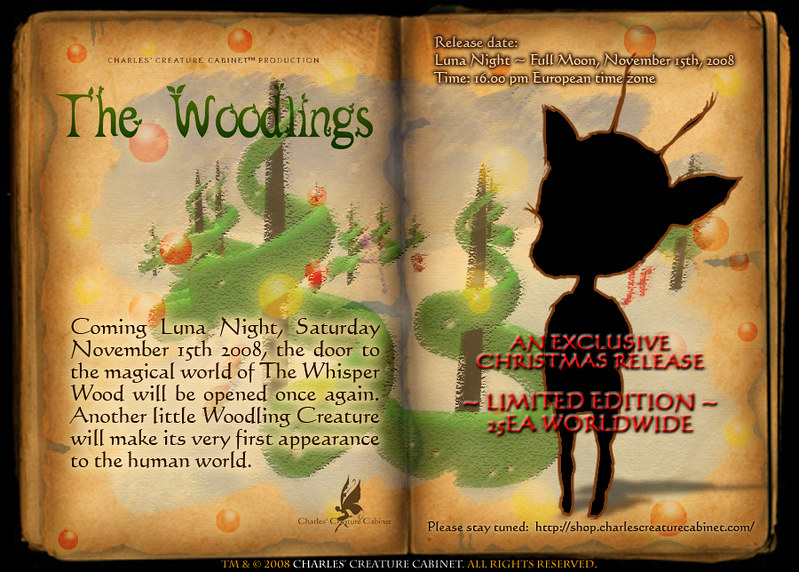This image appears to be an advertisement, likely for a children's book titled "The Woodlings." The scene is reminiscent of vintage parchment with ragged edges, and the design blends snowy hills and spiral-formed Christmas trees decorated with bulbs and lights, all in a palette of greens, golds, and blacks. The top left features green text reading "The Woodlings," and the bottom left segment of the image announces, "Coming Luna Night, Saturday, November 15, 2008: the door to the magical world of the Whisperwood will be open once again. Another woodland creature will make its very first appearance to the human world." This creature is depicted as a silhouetted mystery character on the right-hand side, accompanied by the text "Exclusive Christmas Release, Limited Edition, EA Worldwide." The shadowed figure seems to have the form of a deer with a human-like body, hinting at the enchanting lore of the Whisperwood and adding an element of surprise to this special holiday release. The bottom part of the image contains small, intricate writing, enhancing the overall feel of an ancient, magical manuscript.